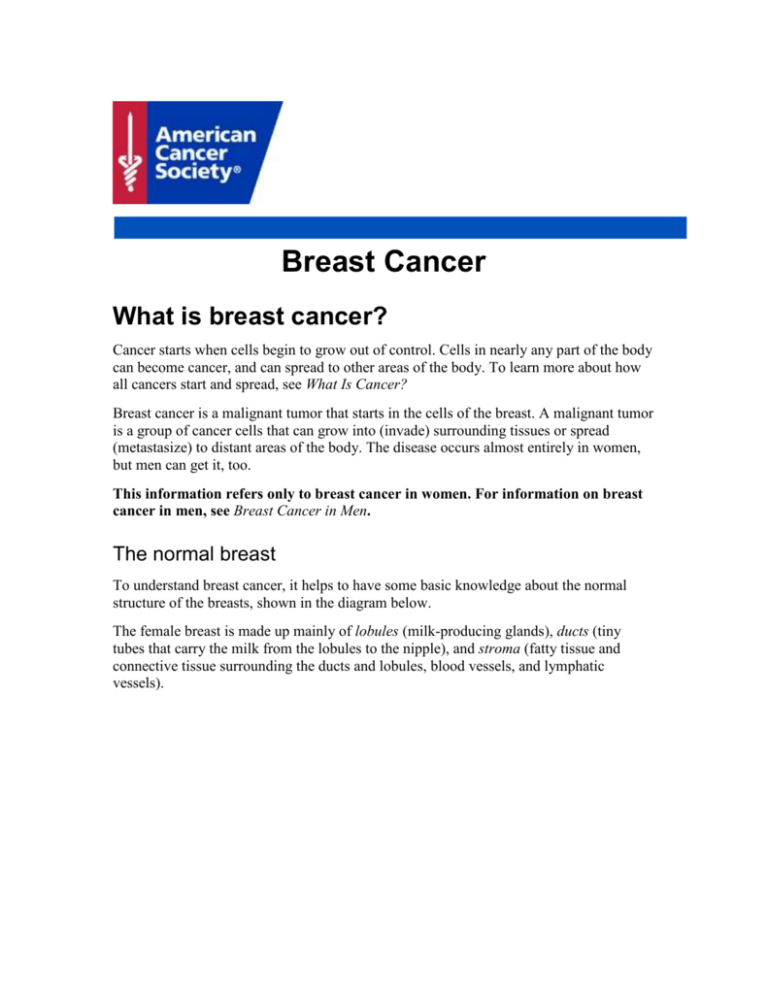**Detailed Caption for the Image:**

The image features a comprehensive informational poster about breast cancer set against a white background. On the left-hand side, there is a distinctive emblem resembling a flag, predominantly red, with a white sword figure within it. Adjacent to the emblem, in a blue section with white text, the words "American Cancer Society" are prominently displayed.

Centered within the poster, there is a noticeable blue bar with bold black text stating "Breast Cancer." Below this, "What is Breast Cancer?" is written in a darker black text. 

The descriptive text provides a detailed explanation of breast cancer, beginning with: "Cancer starts when cells begin to grow out of control. Any part of the body can become cancerous, and it can spread to other areas of the body. To learn more about all cancers and their spread, see 'What is Cancer.'"

Further information elaborates on breast cancer specifically: "Breast Cancer is a malignant tumor that starts in the cells of the breast. A malignant tumor is a group of cancer cells that can grow into and invade surrounding tissue and spread (metastasize) to distant areas of the body. This disease occurs almost entirely in women, but men can get it too." Additionally, it notes, "This information only refers to breast cancer in women. For more information on breast cancer in men, see 'Breast Cancer in Men.'"

To aid in understanding, the text also describes the normal structure of the breast: "To understand breast cancer, it helps to have basic knowledge about the normal structure of the breast, as shown in the diagram below. A female breast is composed of lobes (milk-producing glands), ducts (tiny tubes that carry milk from the lobes to the nipples), and stroma (fatty tissue and connective tissue surrounding the ducts, lobes, blood vessels, and lymphatic vessels)."

This detailed, text-rich poster aims to provide thorough knowledge about breast cancer, emphasizing both the anatomy of the breast and the nature of the disease.